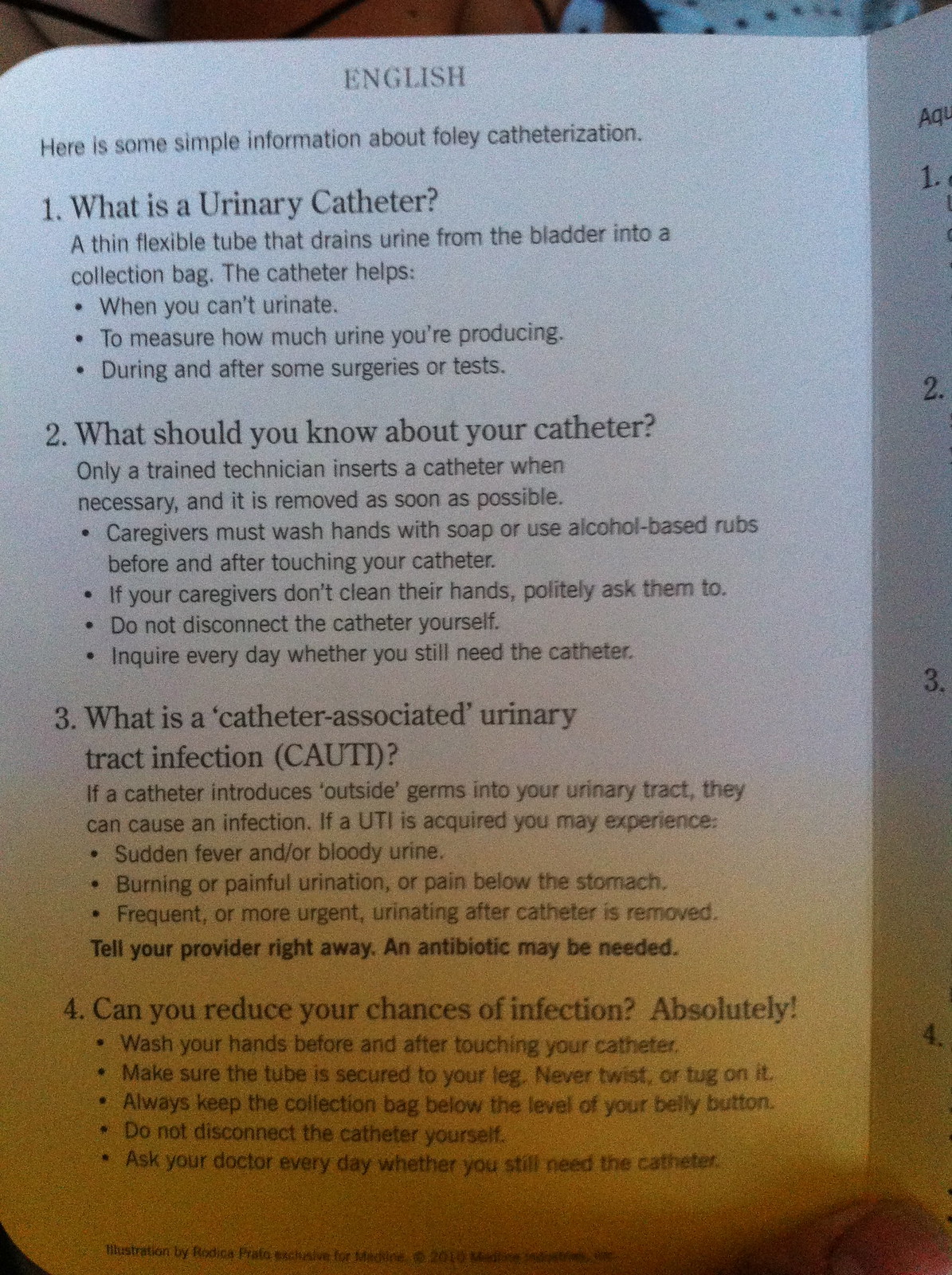This image depicts an informative pamphlet or brochure detailing important information about Foley catheterization. The document, which is presented in English, has a white background with black text and features four main sections. The titles at the top of the pamphlet read: "Here is some simple information about Foley catheterization." Below, there are four numbered bullet points:

1. **What is a urinary catheter?**
2. **What should you know about your catheter?**
3. **What is catheter-associated urinary tract infection?**
4. **Can you reduce your chances of infection? Absolutely.**

Each section includes detailed explanatory text. The first section explains the purpose of a urinary catheter, such as its use when one cannot urinate or to measure urine output during and after surgeries or tests. The other sections provide guidelines and preventive measures to reduce the risk of infection, stressing the importance of actions like consulting your doctor daily about the necessity of the catheter and not disconnecting it by yourself. The pamphlet is well-structured but some parts of the image are slightly blurry due to poor lighting, casting a yellowish shadow at the bottom.